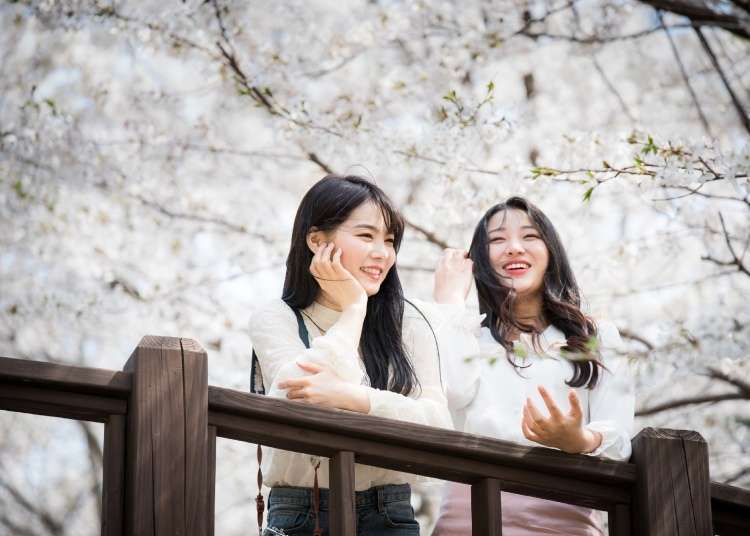The photograph, almost a square but slightly rectangular with the left and right sides shorter than the top and bottom, captures a serene spring day where two young women of Asian descent, appearing to be in their late teens or early to mid-twenties, are leaning against a wooden railing. The background features a pale sky interwoven with tree branches adorned with delicate pale pink blossoms and green leaves. The branches artistically stretch across the top of the image, with a prominent branch in the top right corner extending diagonally downwards, and another significant branch in the lower right, forming a sideways V-shape. Additional thicker branches appear on the lower left, adding depth to the scene.

Both women are dressed in white long-sleeved shirts; the woman on the left is wearing blue jeans and the one on the right is in a pink high-waisted skirt. They are positioned at the center-bottom of the image, with their torsos facing the camera. Their left hands rest on the wooden railing, which varies in height—higher on the left and lower on the right—supported by square-shaped posts. The woman on the right has her right hand in her hair and is smiling with her top teeth showing, looking slightly up. Her slightly wavy hair cascades past her shoulders. The woman on the left supports her cheek and chin with her right hand, looking over to the right. She has a black purse strap over her shoulder, transitioning into a twisted brown strap at the bottom. 

The clarity of the pale, almost white, background and the tender blossoms suggests a setting reminiscent of cherry blossom season in Japan, likely captured within the last 15 years. The women’s expressions of delight and their close interaction, along with the soft, natural color palette comprising whites, browns, blacks, beiges, and pinks, evoke a joyful, conversational moment amidst a picturesque springtime scene.